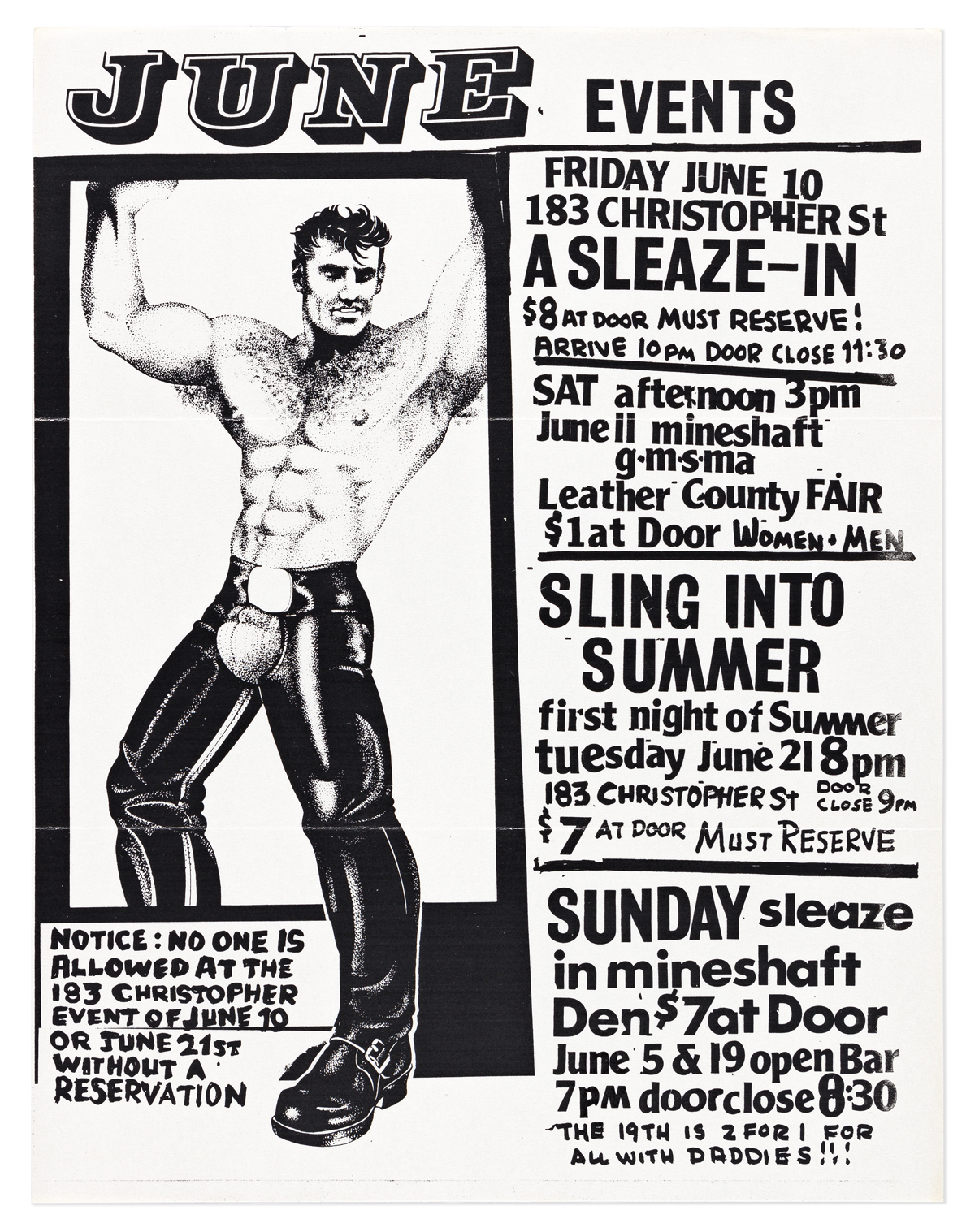This black-and-white poster, likely an old-fashioned advertisement, prominently features the heading "June Events" at the top. On the left side, there's an illustration of a muscular man with short, gelled black hair, shirtless and raising his arms. He sports visible six-pack abs, hairy underarms, black leather pants, and black boots. His cup is worn outside his pants, contributing to the risque tone of the flyer. To the right, detailed event information is listed for June at 183 Christopher Street, including:

- **Friday, June 10th:** "A Sleaze-In," $8 at the door, must reserve, arrive by 10 PM, door closes at 11:30 PM.
- **Saturday, June 11th:** "Mineshaft Leather County Fair," 3 PM, $1 entry.
- **Tuesday, June 21st:** "Sling Into Summer," 8 PM, $7 at the door, must reserve, door closes at 9 PM.
- **Sunday, June 5th and 19th:** "Sunday Sleaze-In Minshaft Den," open bar at 7 PM, $7 at the door, 19th features a two-for-one special with daddies, door closes at 8:30 PM.

Notice emphasizes that reservations are required for several events, and no one is allowed at 183 Christopher Street events on June 10th, 20th, or 21st without a reservation. The poster is filled with black text against a white background, adding to its vintage aesthetic, with each event separated by black lines for clarity.